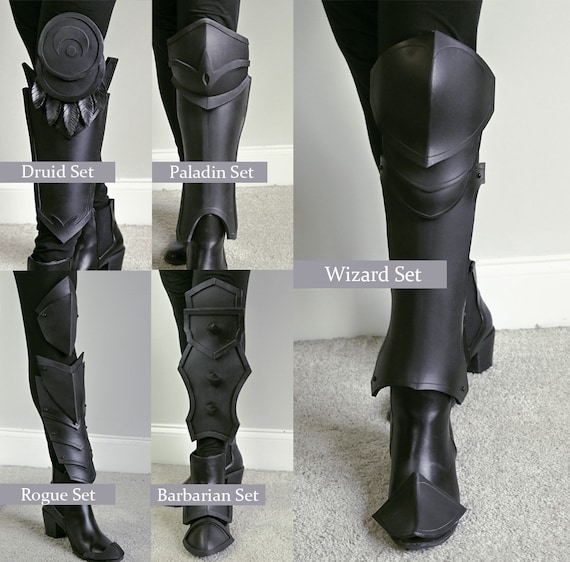The image displays a set of five meticulously crafted leg and foot armor pieces, presumably designed for cosplay or a costume, each modeled on a leg standing on a gray carpet with a light gray wall and white trim in the background. The five photographs are arranged with four smaller images on the left and one larger image on the right. Each set is labeled with a gray bar and white text, denoting common classes from games like Dungeons and Dragons: Druid, Paladin, Wizard, Rogue, and Barbarian. All the pieces are black and 3D-printed, showcasing detailed designs that vary in smoothness and intricacy to correspond with their respective class. 

- The **Druid Set** features feathers sprouting from two circular elements on the top of the boot.
- The **Paladin Set** sports a shield-shaped adornment with an emblem on the upper portion.
- The **Wizard Set** mimics the top of a knight’s helmet with a central ridge.
- The **Barbarian Set** includes a shield-shaped shin guard with three protruding spikes.
- The **Rogue Set** comprises two separate pieces: an upper shin guard shaped like a shield with a central ridge and a lower piece resembling an upside-down triangle.

Each armor set ranges from the toes up to the knee, demonstrating the detailed craftsmanship and thematic consistency in their design.